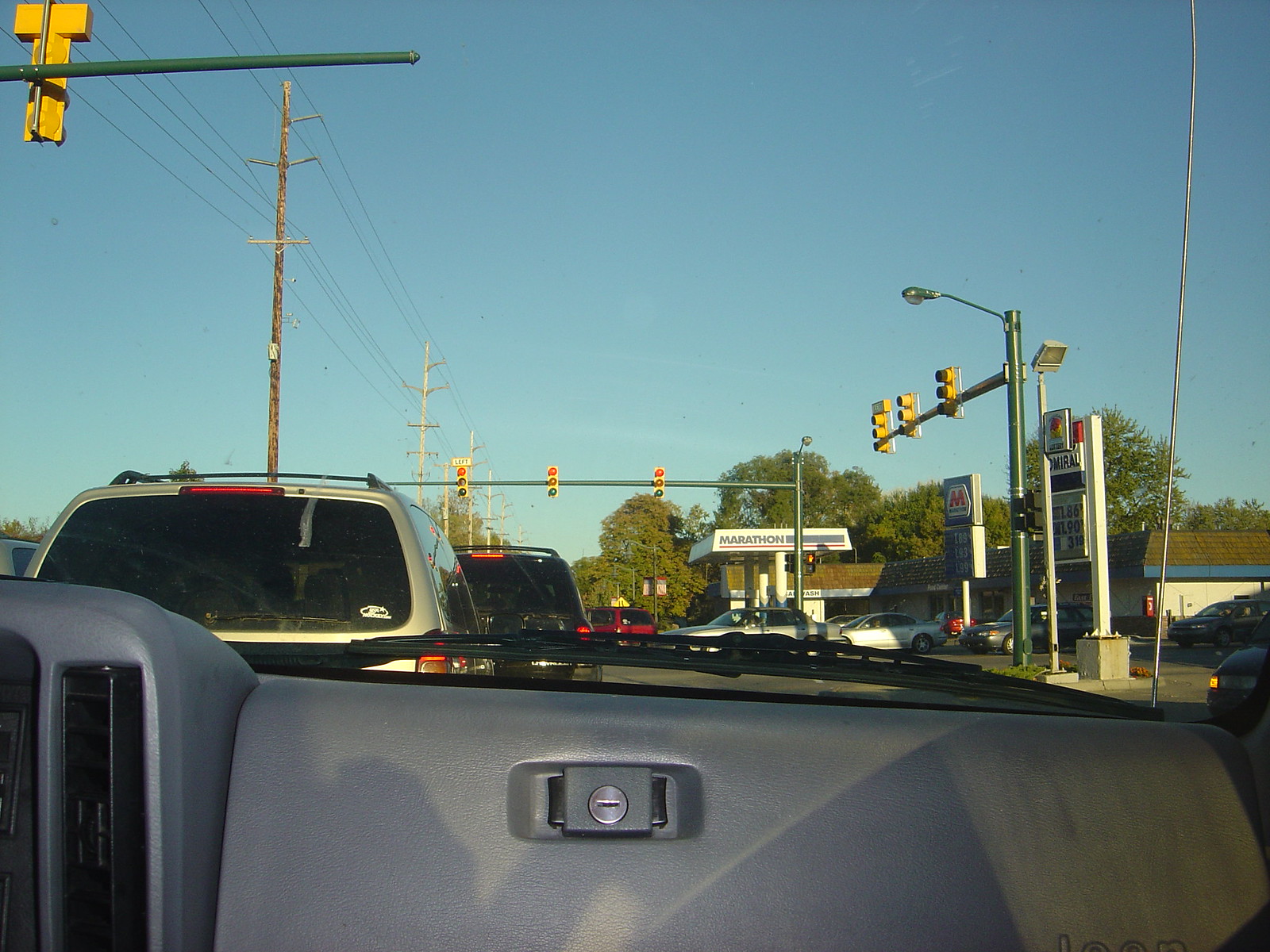This image captures the inside of an older-style car with a black interior. The foreground prominently features the dashboard and the glove box, which appears to have a lock. Through the windshield, a busy intersection stretches out. Traffic is stopped at a red light, with two SUVs ahead—a golden tan one and a black one. The intersection has three traffic lights and three lanes of halted cars while another set of three lanes with a green light can be seen towards the center right. A Marathon gas station with an older-style sign is visible at the center right of the image. The sky is clear, adding a crisp backdrop to the busy urban scene.